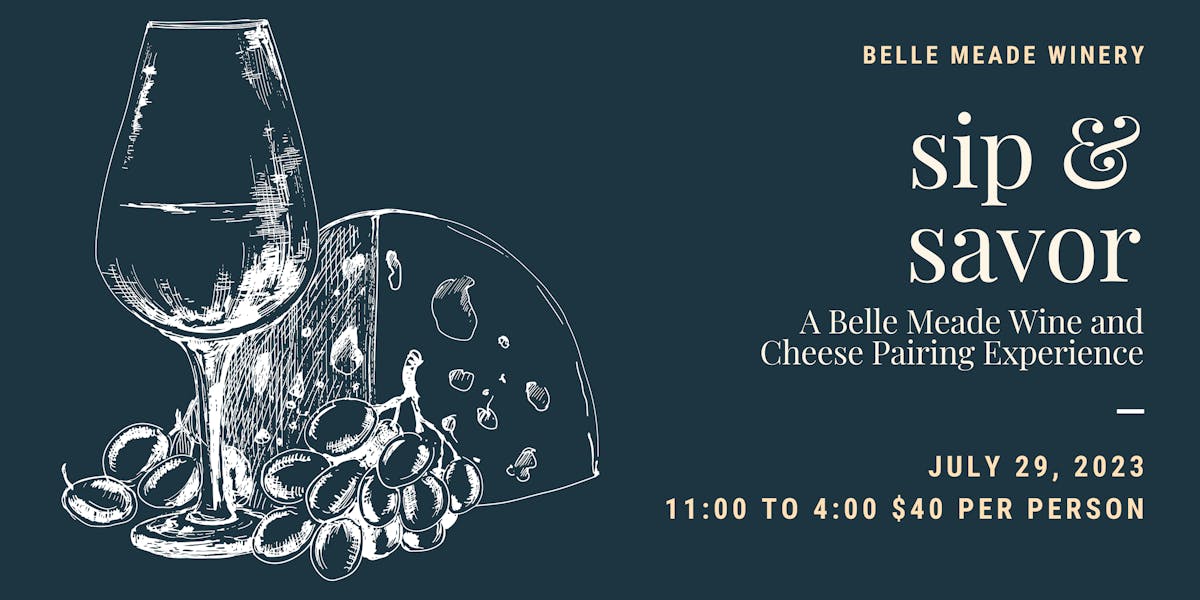This detailed descriptive caption combines and refines the content from all three provided captions:

The image depicts a flyer shaped like a business card, featuring an advertisement for a "Sip and Savor" event at Bell Mead Winery. The background is a deep greenish-blue, almost gray, which contrasts well with the white foreground illustrations. On the left side, white pencil-like sketches depict a wine glass filled with wine, a bunch of grapes, and possibly some cheese. The right side contains the event details: "Bell Mead Winery, Sip and Savor: A Bell Mead Wine and Cheese Pairing Experience, July 29th, 2023, 11 a.m. to 4 p.m., $40 per person." The monochrome design is eye-catching and suitable for both web pages and storefront displays.